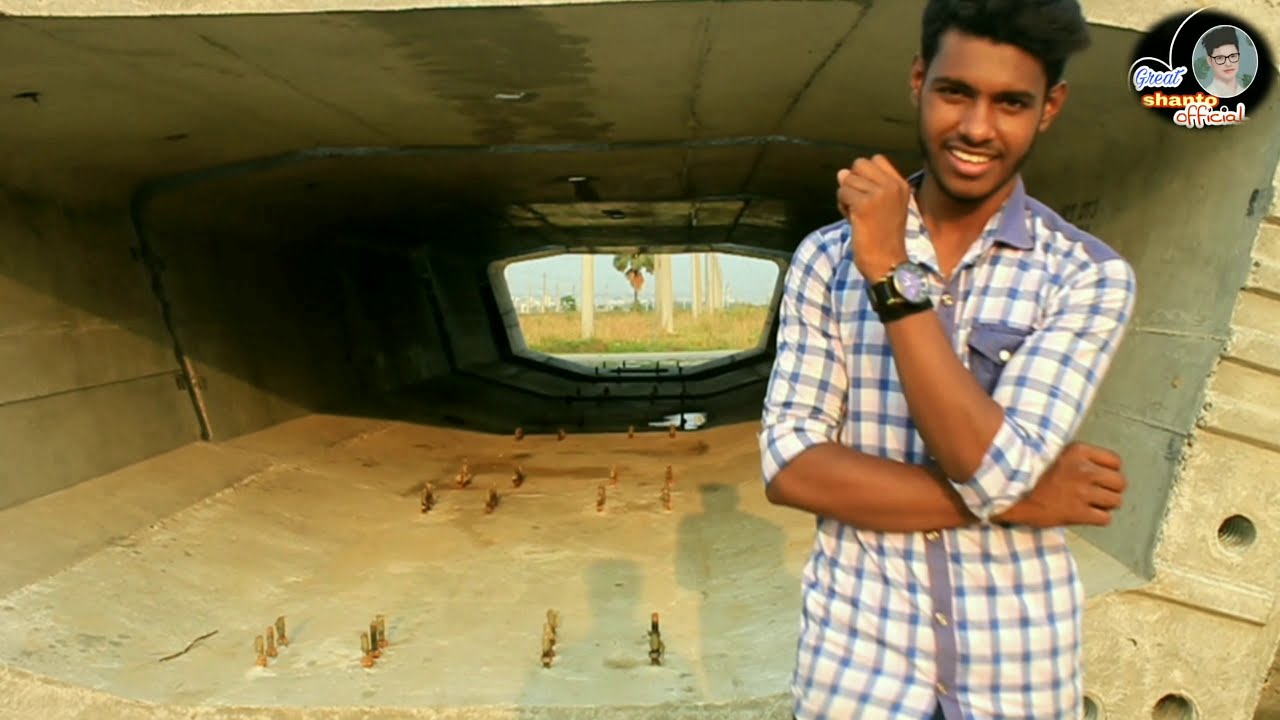In this photograph, a young Indian man, likely in his early to mid-twenties, stands in front of a unique concrete structure that resembles a pentagon-shaped tunnel. He has dark skin, a mustache, and a beard, with tall black hair. The man wears a white button-down shirt featuring blue checks on the collar, shoulders, front pocket, and down the front where the buttons are. His sleeves are rolled up to his elbows, and he sports a black watch on his wrist. He stands with one arm crossed across his belly, the other arm resting on his arm with his fist facing up towards his face, and he is smiling.

The concrete structure he stands before has perfect circular holes at its base and metal spikes arranged in sections. Through the tunnel, one can glimpse a grassy area with green and orange hues, tree trunks, what might be a road or body of water, and white buildings in the distant background against a light blue sky. On the top right corner of the image is a logo, possibly for a YouTube channel or social media, displaying the man's photo. The logo reads "GREAT" in light blue, "SHANTO" in orange, and "OFFICIAL" in red letters. Shadows of two people are faintly visible in the forefront within the structure.